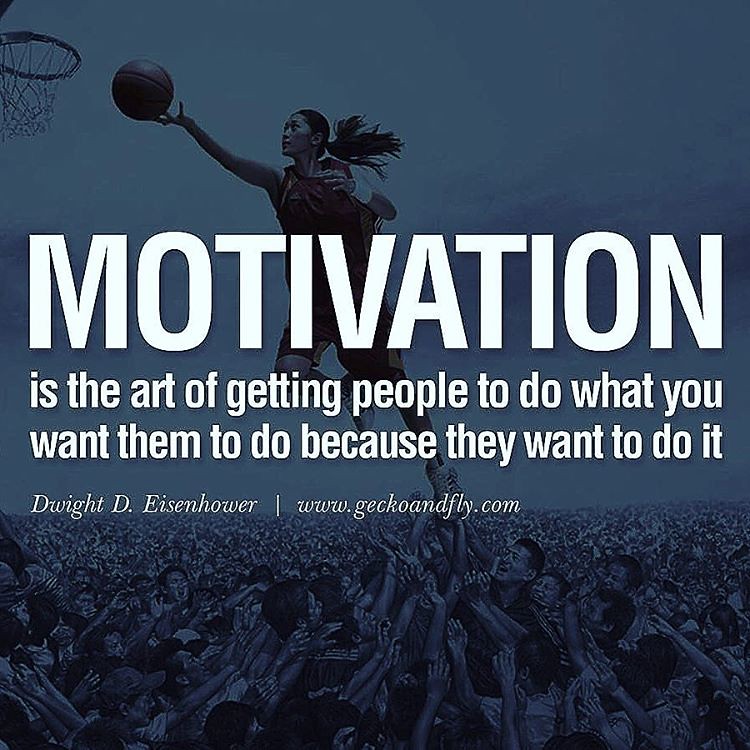This square, motivational graphic features a dynamic image of a woman making a high-flying layup towards a basketball hoop in the top left corner. Her fit and athletic figure, with a ponytail streaming behind her, is elevated in mid-air, seemingly propelled by a crowd of people below, their arms raised to support and hoist her up. The background is washed with a dark blue filter, adding a striking contrast to the scene. Dominating the image from left to right is the bold, white sans serif text "MOTIVATION." Below this, in smaller bold white lowercase letters, is the quote, "is the art of getting people to do what you want them to do because they want to do it," attributed to Dwight D. Eisenhower. Justified to the left and italicized in serif font, the name "Dwight D. Eisenhower" is followed by a vertical bar and the website "www.geckoandfly.com."